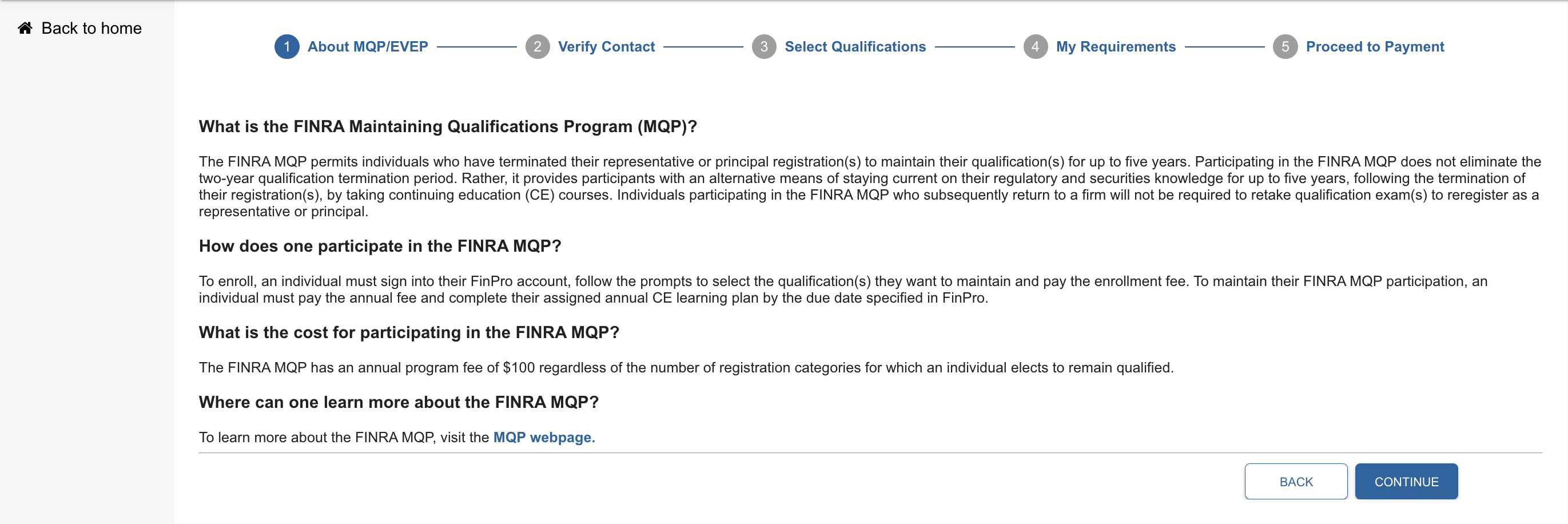The image is a screenshot with a white background and a light gray horizontal border at the top. Below the border, a navigation guide is presented from left to right in blue text. The steps are outlined as follows: 

1. "About MQP/EVEP."
2. "Verify Contact" within a gray circle.
3. "Select Qualifications."
4. "My Requirements."
5. "Proceed to Payment."

Beneath this sequence, bold black text asks, "What is the FINRA Maintaining Qualifications Program (MQP)?" Following this, smaller gray text explains that "The FINRA MQP permits individuals who have terminated their representative or principal registration to maintain their qualification for up to five years. Participating in the FINRA MQP does not eliminate the two-year qualification termination period."

In the lower right corner of the screenshot are two action buttons. The left button is white with blue text that reads "Back," and the button to the right is blue with white text that reads "Continue."